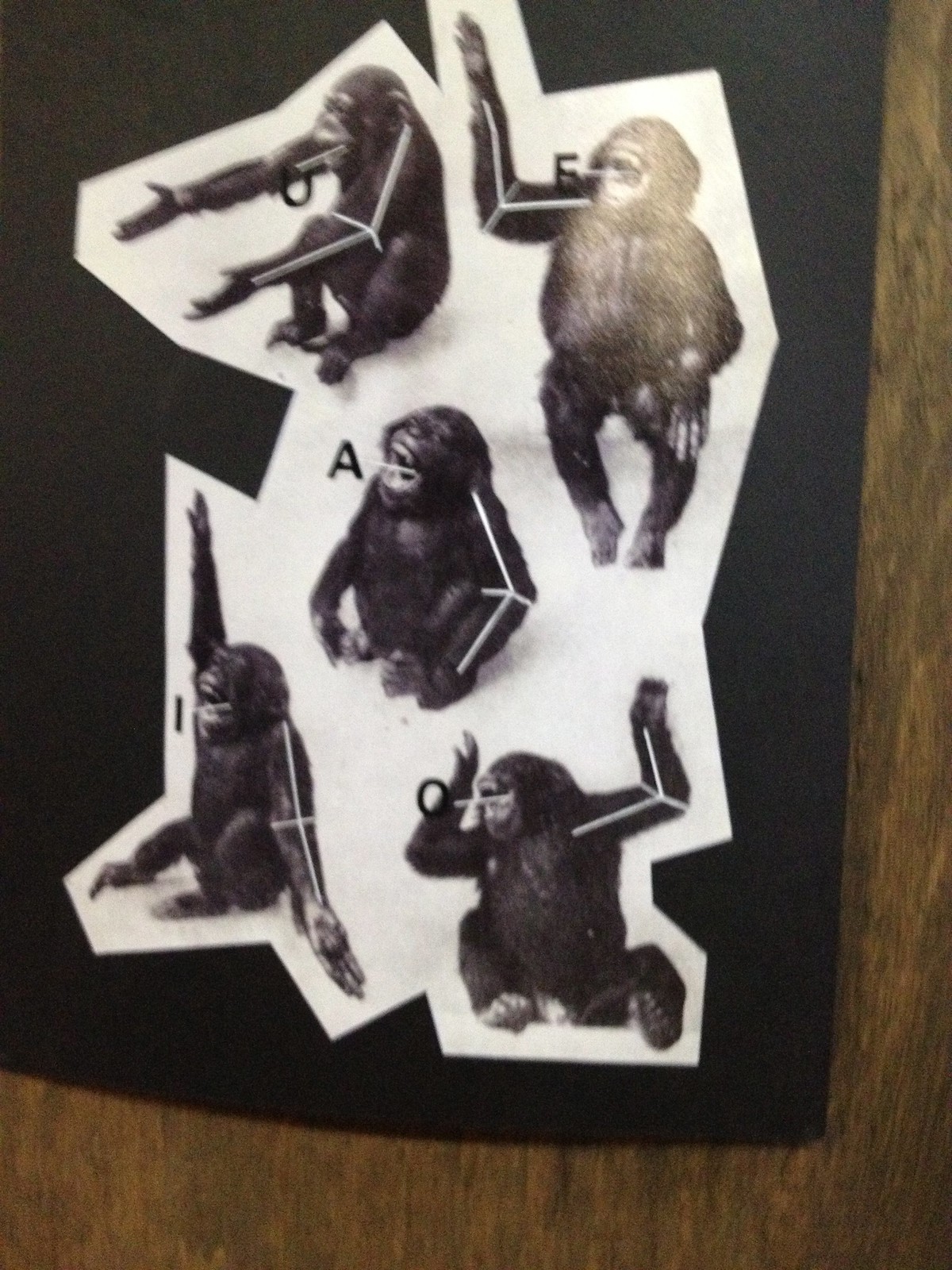This image is a photograph of a collage featuring five distinct photographs of the same small chimpanzee, each in different positions, pasted onto a jagged, irregularly cut white paper. This white paper is mounted on a black background, which itself is placed against a wooden surface, possibly a door or wall. The chimpanzee images appear to be demonstrating various shapes or symbols, each labeled with a letter: A, E, I, O, and U. White lines on the chimpanzee's arms highlight their positions, suggesting an educational or communicative purpose. The overall layout resembles a poster or visual aid, illustrating the different ways the chimpanzee can form the specified letters through its gestures.